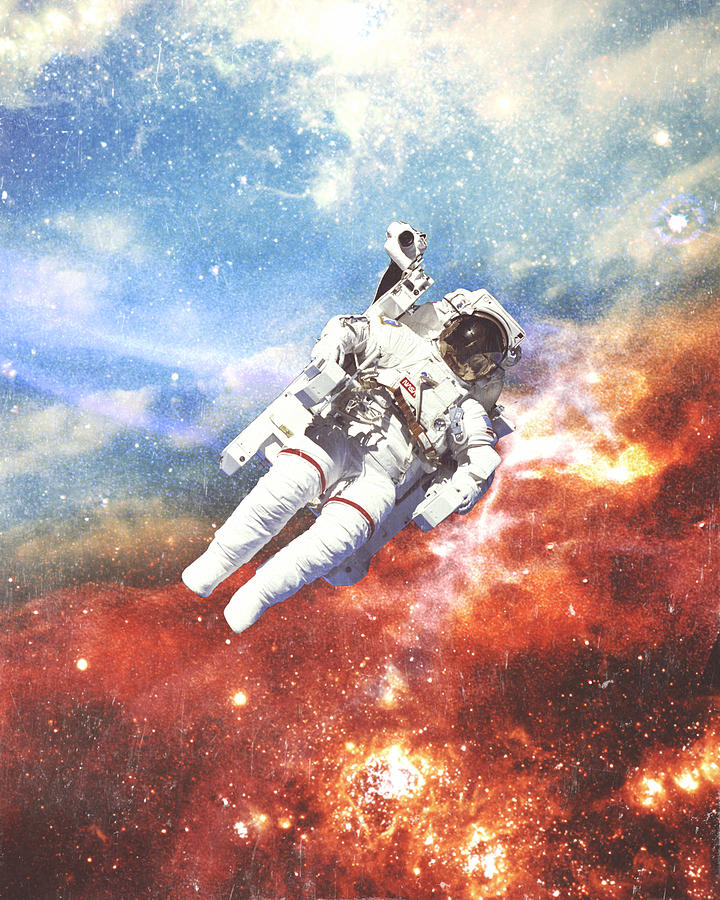This vertical rectangular painting depicts an astronaut in a white suit, floating at a tilted angle with his head aligned toward the top right corner and his feet down toward the bottom left corner. The astronaut's face is obscured by a dark helmet, and he has a camera mounted on a jetpack strapped to his back. The background is a vibrant, tie-dye-like cosmic scene, with the top half featuring a bluish sky with clouds and many stars, while the bottom half transitions to dark space with swirling red and white clouds, punctuated by more stars and galaxies. The division between the blue and red hues of the background runs diagonally, mirroring the angle of the astronaut's body.